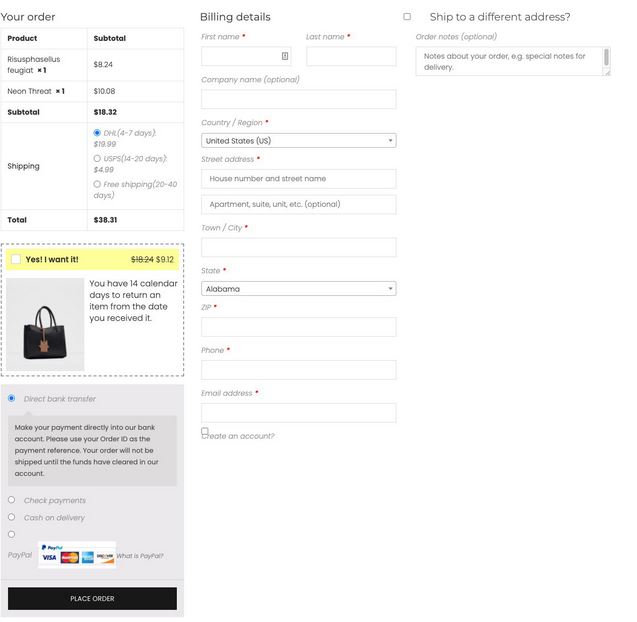This image is a screenshot of an online purchasing screen, detailing the checkout process for a customer. Starting at the upper left-hand corner, the "Order Summary" section shows that the customer is purchasing an item named "Risu Vasilis Fugiat" priced at $8.24 and another item called "Neon Threat" costing $10.08. The subtotal for these items is calculated at $18.32. The customer has selected DHL 4-7 day shipping, which adds an additional $19.99 to the cost. Consequently, the total purchase amount sums up to $38.31.

Below the order summary, there is an option to add a handbag to the order for $9.12, but the customer has not chosen this item. The selected payment method is a direct bank transfer. However, the customer's billing details remain incomplete. Required fields including the first name, last name, and optional company name, as well as country/region and the street address (with room for additional optional information like apartment/suite/unit), have not been filled out. Town/city details are also missing, though the customer has selected Alabama as their state. The zip code, phone number, and email address fields are blank.

On the right side of the screen is an option asking if the customer would like to ship to a different address, but this option is currently unchecked.